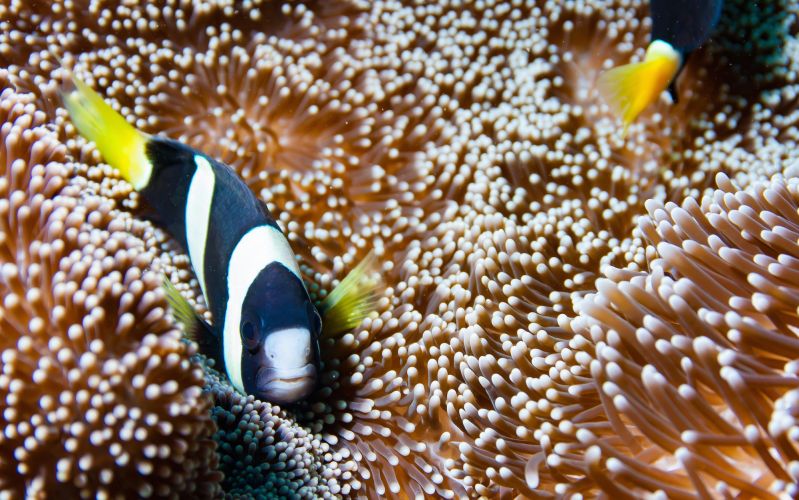This is a detailed color photograph showcasing a clear underwater scene, potentially a saltwater fish tank or the ocean. Dominating the composition, we see a pair of black and white striped fish, often reminiscent of clownfish, with distinct yellow fins and bright yellow tails. The fish on the left, with its white nose and black eyes, is directly facing the camera, capturing our attention. The other fish, partially cropped and visible in the upper right, reveals only its black-striped body and vibrant yellow tail. Both fish swim amidst an underwater anemone, which features hundreds of brown tube-like arms with white tips, resembling Q-tips. The anemone's appendages appear to sway gently, enhanced by the photo's slightly muted colors and the ambient light illuminating from the left side. The light source suggests possible origins, such as an ROV or a diver, although the scene itself doesn't seem very deep. Overall, the photograph adeptly captures the serene beauty and intricate details of this underwater moment.